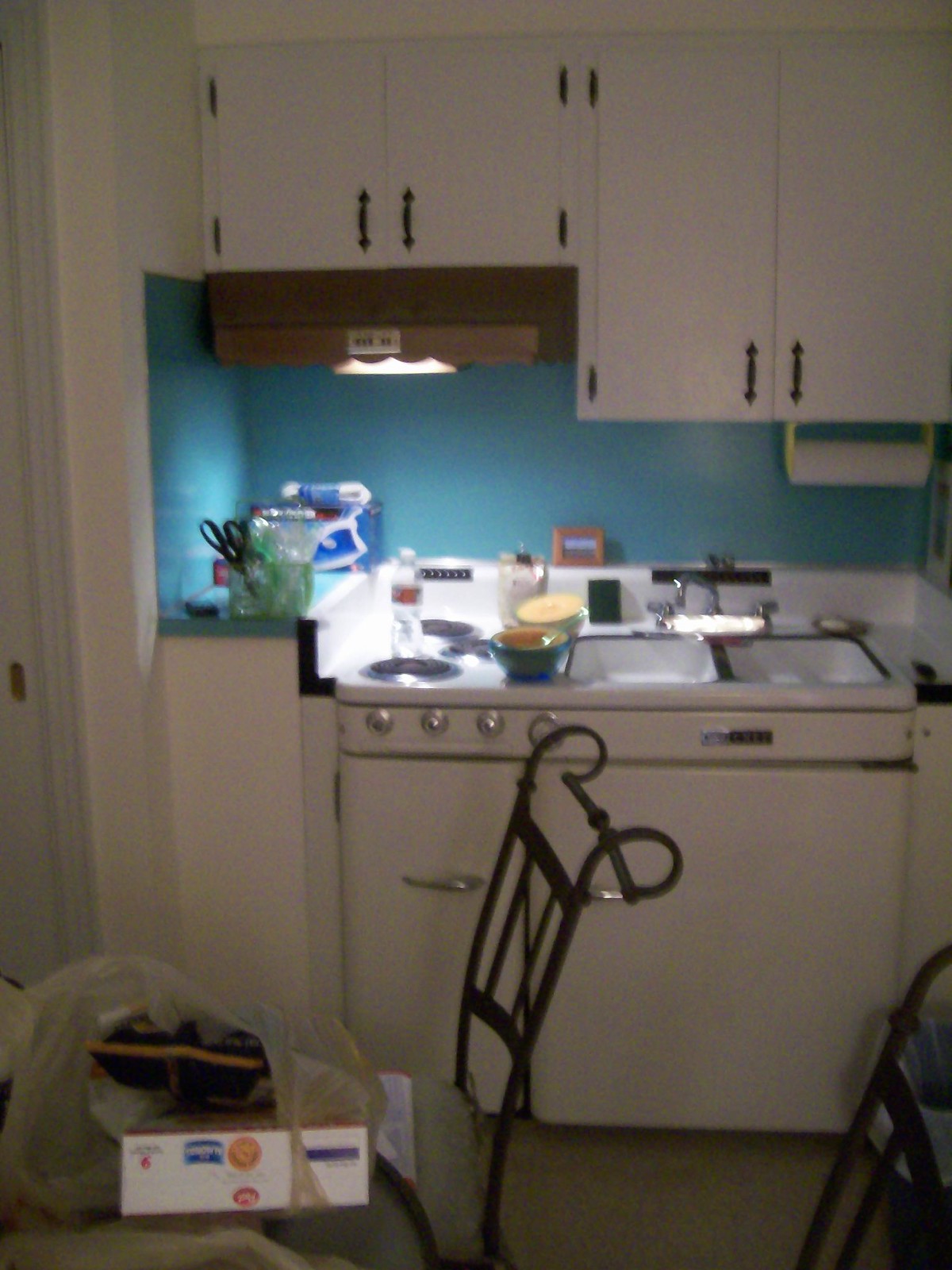The image depicts a slightly cluttered kitchen. On the left, a white doorway leads into the scene, followed by a beige countertop with a teal-colored backsplash. A narrow white stove, likely with three elements as indicated by the three dials, is partially obscured by a water bottle resting on it. To the right of the stove, a small double-basin sink is integrated into a white countertop. A bar of soap is situated in the upper right corner of the sink area. 

Above the stove, a wooden light fixture is attached to the white cabinets adorned with black handles. 

In the foreground, there is a table that appears to hold a bag of groceries, accompanied by two wire chairs. The chairs have intricate wiring designs at the tops of their backs, adding a touch of detail to the slightly chaotic, yet homey scene.